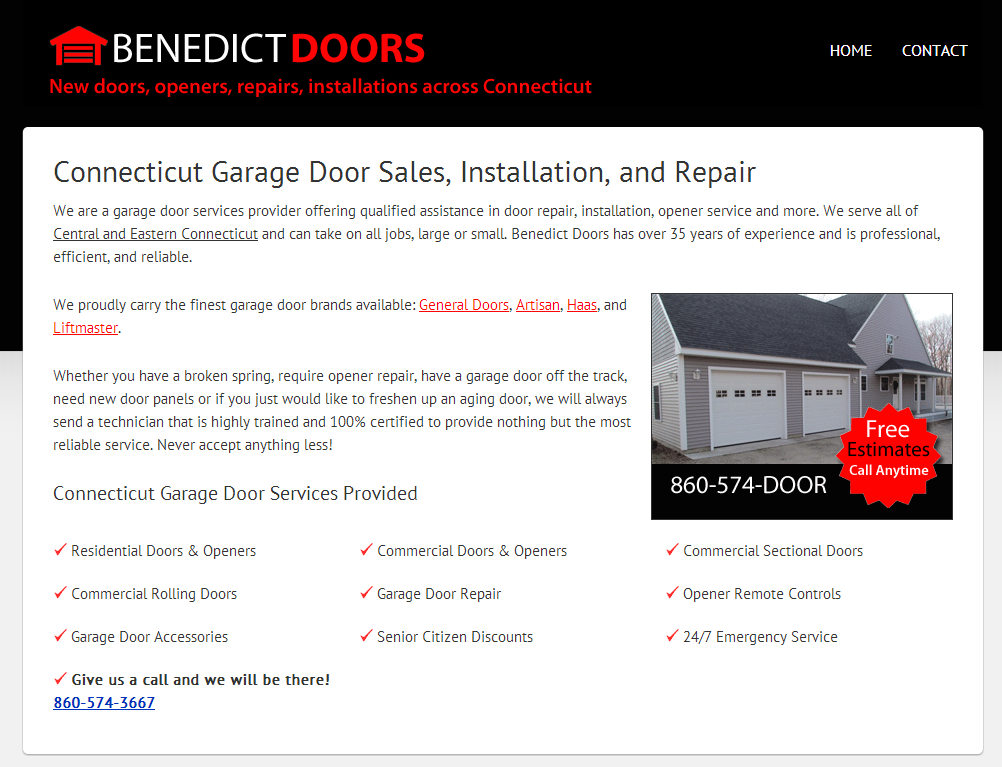Cropped screenshot of the Benedict Doors website. The top left corner features a black background with the company name, "Benedict Doors," and a garage door logo. Below this, in red text, the services listed are "New Doors, Openers, Repairs, Installations across Connecticut." On the top right, white text provides navigation links for "Home" and "Contact."

Dominating the page is a large white box, set against a black upper half and grey lower half of the webpage. This box bears the header "Connecticut Garage Door Sales, Installation, and Repair" in bold black letters. Underneath, a detailed company description is provided. The center section highlights the brands offered, stating, "We proudly carry the finest garage door brands available, including General Doors, Artisan, Haas, and LiftMaster," with each brand name hyperlinked in red.

At the bottom of the page on the left, a blue hyperlinked telephone number can be found. Toward the center-right, there is a thumbnail image of two garage doors attached to a house, alongside another telephone number. A sticker in the bottom right corner of the thumbnail reads, "Free estimates, call anytime."